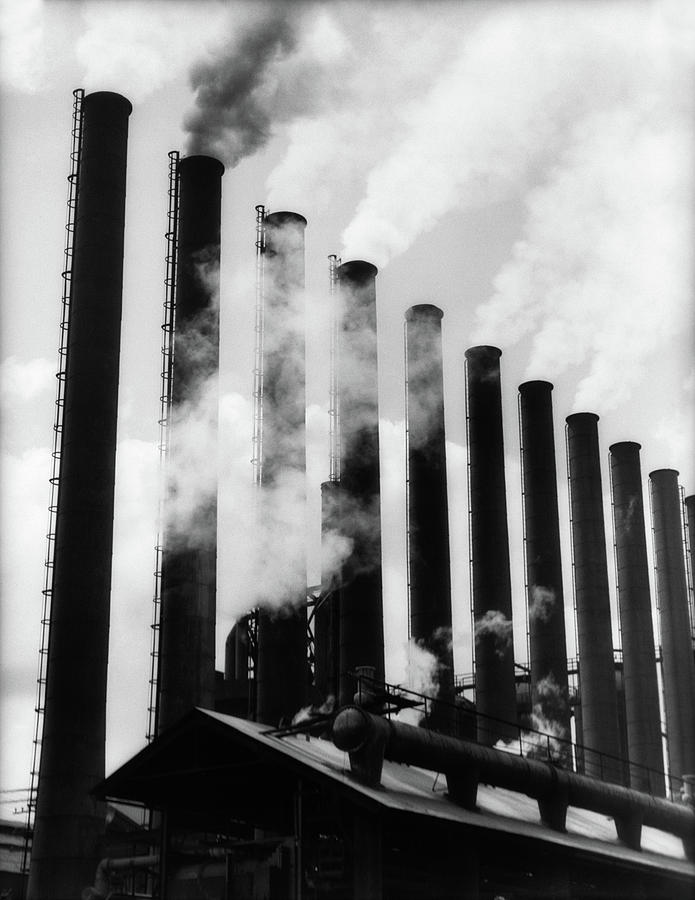The image is a historical black and white photograph of an industrial factory scene dominated by numerous tall smokestacks, with a total of at least 11 visible. Each smokestack is equipped with a metallic ladder climbing up its side, presumably for maintenance purposes. The smokestacks are uniformly emitting smoke of varying shades; most are releasing white smoke, but the second stack from the left is notable for its darker, black smoke, indicating potentially heavy pollution or a malfunction that may need checking. A large black building or structure with a tin roof is visible at the bottom of the image, and it features a thick black pipe running along the roofline. The sky overhead is a uniform shade of grey, blending seamlessly with the smoke and adding to the overall industrial and somewhat grim atmosphere of the scene. There are no people or the sun visible in the image, emphasizing the stark and mechanical nature of the factory setting.